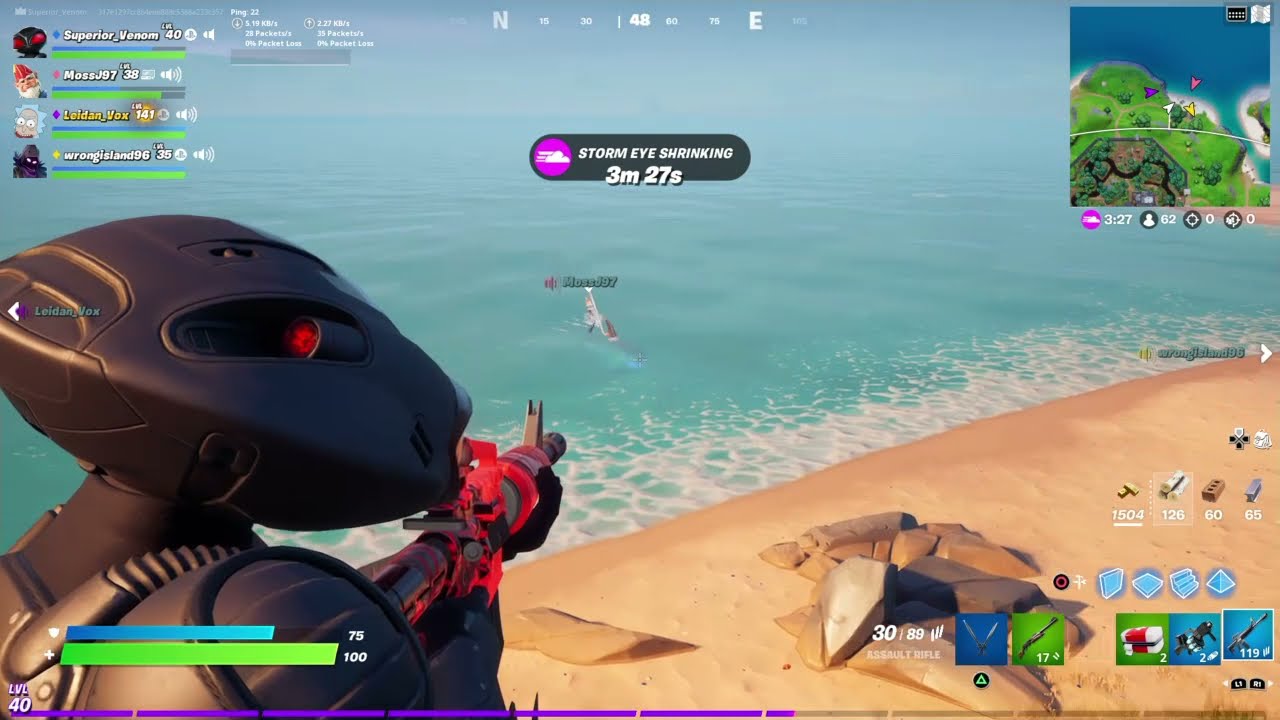This is a detailed screenshot from the video game Fortnite, showcasing a scene from a third-person perspective. The player’s character is outfitted in the Black Manta skin from the Aquaman series, distinguished by its dark gray, metallic humanoid appearance and long, cylindrical head. The character is wielding a striking red assault rifle, aimed towards the ocean from the shoreline. The water close to the beach has a greenish tinge, contrasting with the softer blue of the distant waves. In the water, directly in the line of the gun, is an indistinct figure, possibly the target.

The upper right-hand corner of the screen features a mini-map, indicating the local geographical context with an island, beach, and ocean. Just to the right of the character's head, a notification reads, "Storm Eye Shrinking 3 minutes 27 seconds," signifying an impending game event. Below the mini-map, in the corner, are green and blue health bars, alongside icons representing different weapons and ammunition counts.

On the left side of the screen, several statistics and player scores are displayed, with notable names like "Superior Venom" accompanied by scores. The top center of the screen includes a compass bearing, reading 48 degrees, indicating the direction the character is facing. Overall, the screenshot vividly captures a moment of in-game action and player status within Fortnite’s dynamic environment.